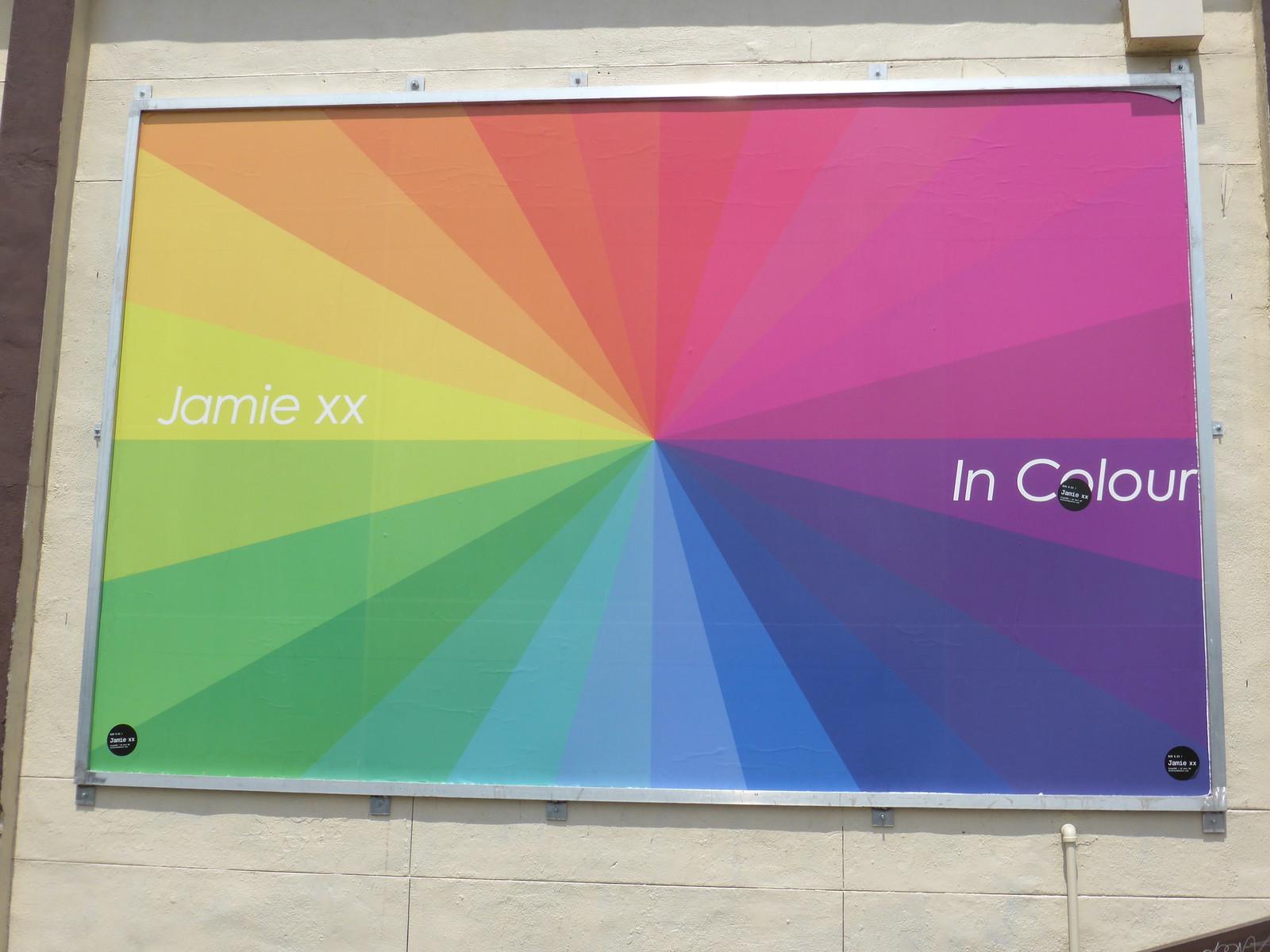The image is a rectangular sign under construction, set against a beige background reminiscent of the back of a frame. Central to the sign is a metallic frame with multiple screw holes designed for mounting. Inside the frame, the sign features a vibrant color wheel displaying a full spectrum of hues.

Starting from the top, at the 12 o'clock position, the wheel showcases reds transitioning into magentas. As it moves clockwise to the 3 o'clock position, the colors shift into purples and blues. Continuing the circular gradient, the lower-left section, around the 6 o'clock position, features greens, which then blend into yellows as they reach the 9 o'clock mark. The sequence completes with oranges leading back up to the reds.

Text elements punctuate this colorful arrangement. On the left side, within the green-yellow sector of the wheel, the word "Jamie" is inscribed in lowercase letters followed by "xx." On the opposite side, within the purple segment, the words "in color" are displayed. 

Additionally, there are three small black dots with inscriptions: two are situated on the right side, and one is located in the lower left corner. These dots contain further details, though their specific wording is not clear.

Overall, the sign harmoniously combines text and color within a robust metallic structure, suggesting an artistic piece in the midst of creation.